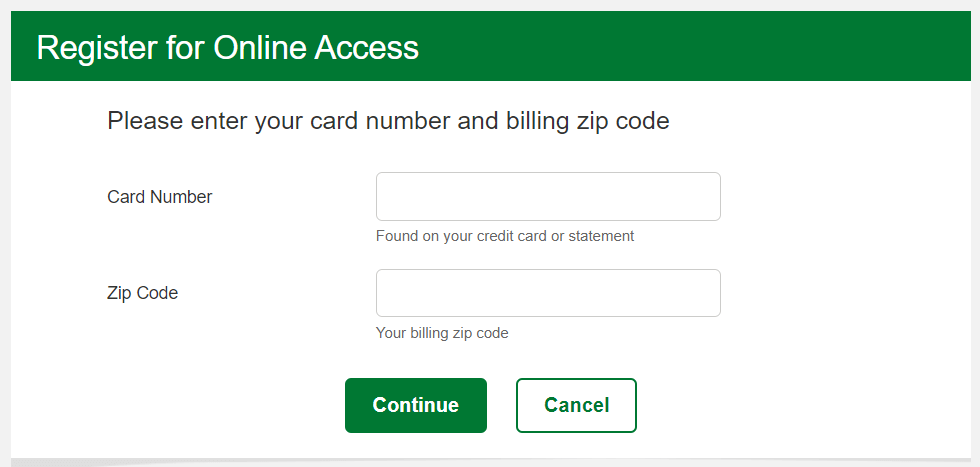The image is a screenshot from a website, divided into two distinct sections. The top 10-15% of the screenshot features a blue bar with white text that reads "Register for Online Access" against a plain green background. The remaining 80% of the screen is predominantly white, featuring two input fields. Above these fields, a prompt in bold text asks the user to "Please enter your card number and billing zip code."

The first input box is labeled "Card Number" on its left side, with a horizontally-aligned, elongated text area where users can enter their card details. Beneath this box, a helpful hint states that the required information can be "found on your credit card or statement."

The second input field, positioned directly beneath the first, is labeled "Zip Code." Below this text box, there is a hint reminding users to enter their "billing zip code."

At the bottom of the input section are two buttons. The first button, labeled "Continue," is a green rectangle with white text. To its right is the "Cancel" button, which features a white background with a green border, with the word "Cancel" displayed in green font. This button setup contrasts the green continue button and the white cancel button, reinforcing the primary action.